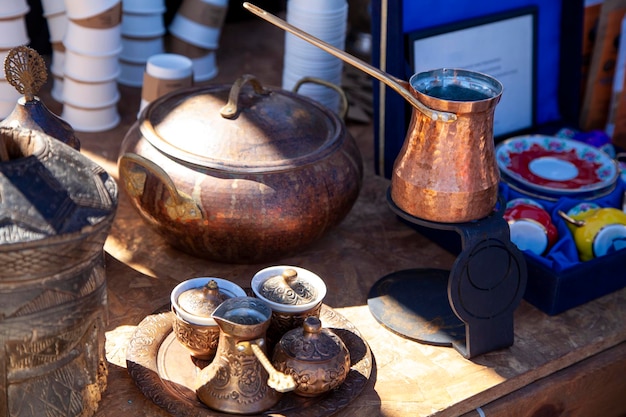The image depicts a scene reminiscent of a traditional tea or coffee brewing station, possibly inspired by Turkish or other Middle Eastern styles. Central to the image is a large copper kettle with side handles and a lid, situated on a wooden surface. Surrounding the kettle is a collection of smaller copper and brass containers, including pitchers and sugar holders, all fitted with lids. The setup also features a distinctive black contraption with a circular base and extended back piece, topped by another copper container with a long handle, likely used for brewing. To the side, there are several white and red bowls, along with an array of paper coffee cups, suggesting a beverage station. In the background, stacks of white cups with brown accents are visible, adding to the impression of a well-organized tea or coffee service area.